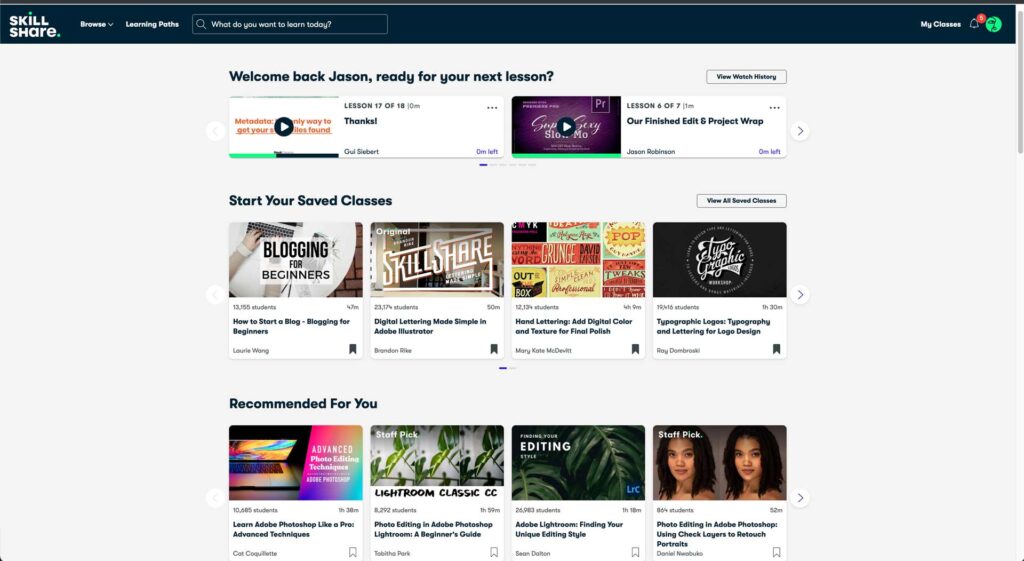The image showcases a well-organized dashboard on the Skill Share platform. In the upper left corner, the logo "Skill Share" is displayed prominently, with "Skill" positioned above "Share." Adjacent to this are options labeled "Browse" and "Learning Paths."

The central section of the dashboard greets the user with a friendly "Welcome back, Jason. Ready for your next lesson?" Four video thumbnails are lined up horizontally, two of which feature play arrow icons indicating they are videos. One of these thumbnails has a partially filled green progress bar beneath it, while the other has a fully filled green progress bar.

Below this row, the section "Start Your Saved Classes" is visible, displaying an image of a person typing on a laptop on a white table with the course title "Blogging for Beginners." Beside it, the Skill Share logo is shown again, along with two additional class thumbnails.

At the bottom of the dashboard, under "Recommended for You," there is an array of class suggestions. The first thumbnail depicts a laptop with a multicolored screen in shades of pink, yellow, and blue. The next image shows green plants on a screen, followed by another thumbnail with a dark green background and green plants titled "Editing" in white text. The final thumbnail features a woman with short dark hair, displayed twice, with a label "Staff Pick" on it.